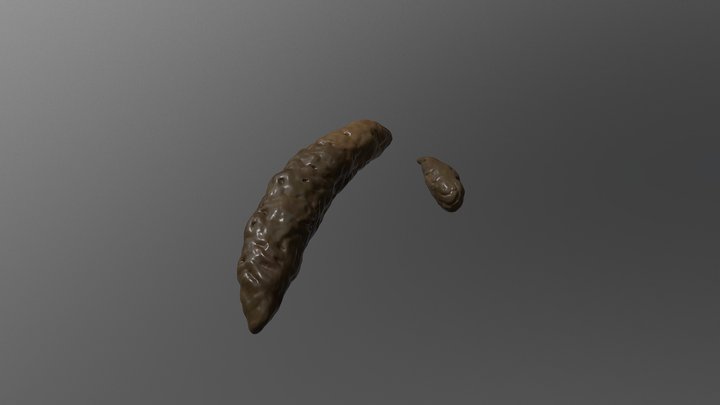This horizontally rectangular photograph features a gradient gray background that transitions from lighter gray in the upper left corner to darker gray in the bottom right. At the center of the image, two brown, tube-shaped objects are prominently displayed. The larger object on the left has an elongated form with a dark brown hue, filled with holes that give it a textured, porous appearance. The smaller object on the right is pea-sized and seems to be made of the same material as the larger one. Both objects bear a striking resemblance to feces, though they could potentially be ceramic models or minerals, given their reflective, shiny surface. The image appears to be taken under artificial lighting, enhancing the contrast between the objects and the gradient background.